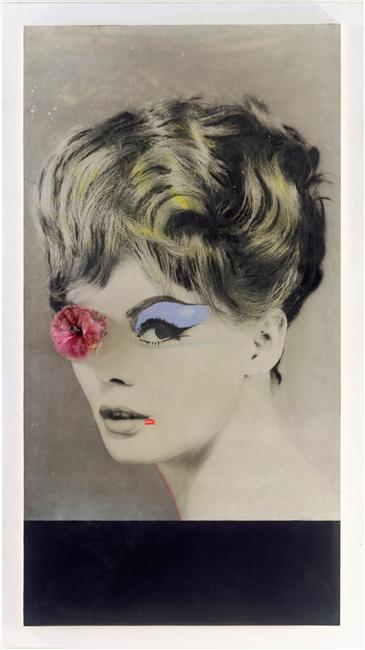The image is a striking photograph-turned-pop-art of a woman with a distinctive 1950s hairstyle, reminiscent of the rebellious era of motorcycle clubs and beatnik culture. She sports a bob haircut with finely penciled high-arched eyebrows, heavy winged eyeliner, and false eyelashes that accentuate her vintage look. Her makeup is distinctly stylized with a heavy blue eyeshadow applied over one eye, while a vibrant red flower covers her other eye, creating a vivid focal point. The image is meticulously detailed, including a small red mark near her slightly open lips and her long neck, as she gazes to the left with an enigmatic expression. The photograph is framed with a dark black border at the bottom, devoid of any artist’s signature or text.